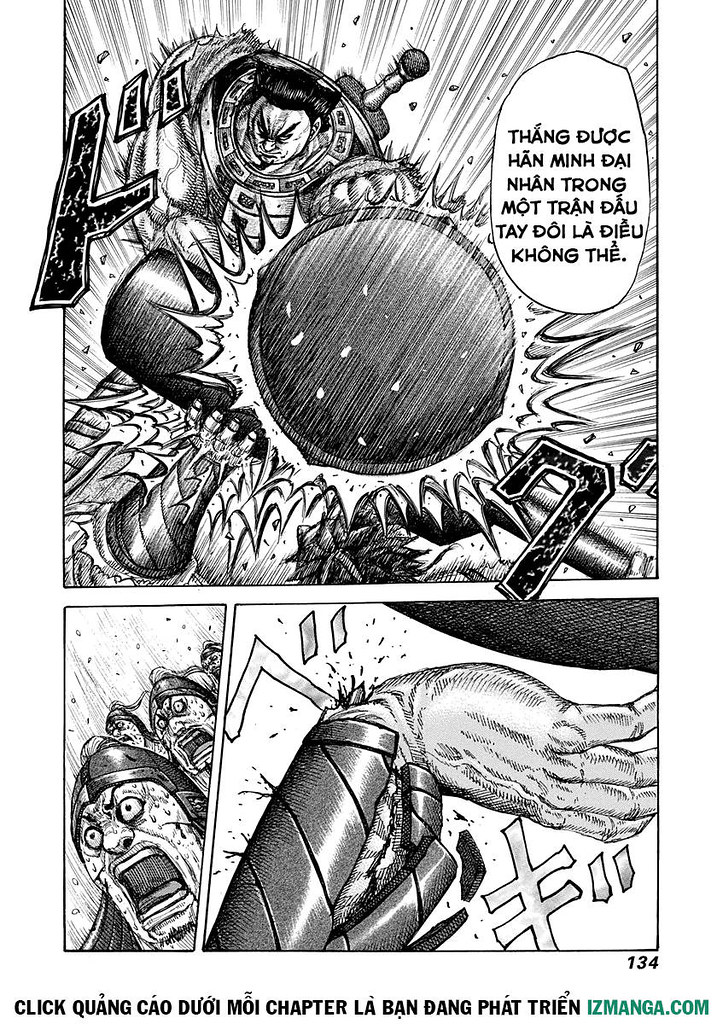The comic strip is depicted in black and white and consists of three segments. The top segment is a large square panel portraying a dramatic scene with strong action lines. It features a man, possibly a villain, dressed in samurai-like armor with spiky black hair. He appears to be attacking with a shield held out in front of him, accompanied by a text bubble written in a foreign language. Beneath this main panel, the comic strip is divided into two asymmetrical rectangles. The panel on the lower left shows a chaotic scene of several men in helmets, their faces contorted in fear as if reacting to something falling upon them, indicated by numerous action lines. The final panel on the right depicts a gruesome close-up of a hand holding up a shield, with the wrist bending unnaturally backward, suggesting the bone has broken from the force of the impact. This striking imagery underscores the intensity and violence of the encounter.